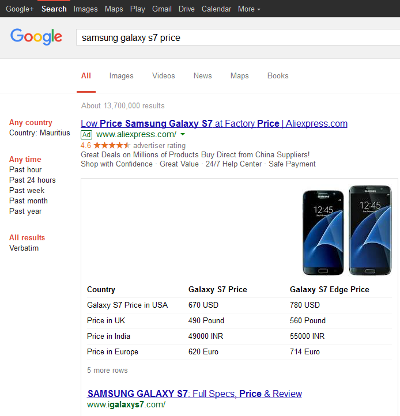The screenshot features a Google search result page with the search query "Samsung Galaxy S7 price" entered in the search bar. The image quality is notably low, making text difficult to decipher. The search page displays the Google logo and standard search bar at the top, with tabs for All, Images, Videos, News, Maps, and Books. The "All" tab is currently selected. On the left-hand side, there's a column listing various filter options: any country, anytime (with sub-options past hour, past 24 hours, past week, past month, past year), all results, and verbatim. The search query returns approximately 13,700,000 results.

The first search result is an ad from aliexpress.com, advertising "low price Samsung Galaxy S7 at factory price" with a 4.6-star rating. The ad highlights great deals on millions of products directly from China suppliers, emphasizing the benefits of shopping with confidence, great value, a 24-7 help center, and safe payment options.

The second result is from the website igalaxyss7.com, titled "Samsung Galaxy S7 Full Specs Price and Review." This entry includes an image of the Galaxy S7 Edge and provides pricing information for both the Galaxy S7 and the Galaxy S7 Edge, along with the respective prices in different countries.